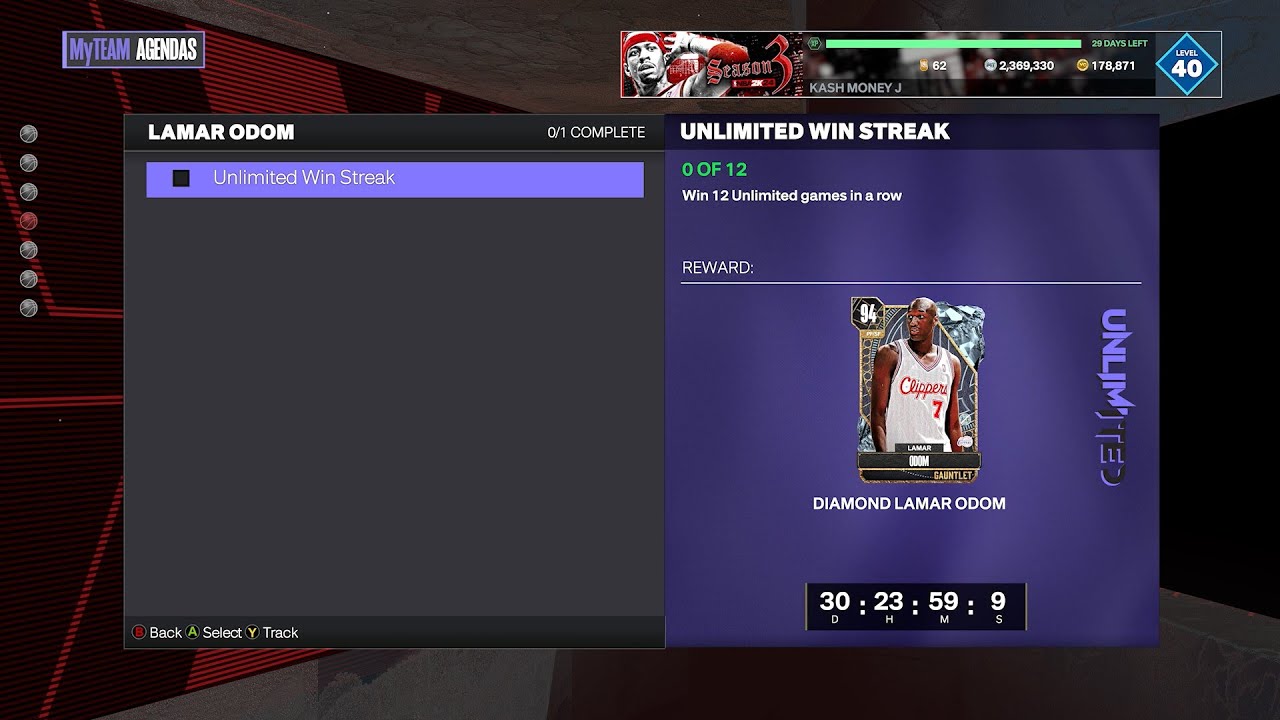The image is a screenshot from a basketball video game, featuring a user interface related to team progress and challenges. In the top left-hand corner, there's a purple box labeled "MY TEAM AGENDAS" in white uppercase letters, with "TEAM" prominently in all caps. The background appears to display part of a basketball court or a room with dark red stripes on the left-hand side. In this area, several basketballs are arranged vertically; most are gray, with a notable orange basketball in the middle.

Towards the center, there's a dark gray rectangle highlighting a specific task related to Lamar Odom. The text reads "Lamar Odom" at the top, with "0 out of 1 complete" beneath it. A highlighted purple box notes the task "Unlimited win streak," with buttons labeled "back," "select," and "track" at the bottom.

On the right side of the image, another purple box titled "Unlimited Win Streak" provides details for a challenge: "Win 12 unlimited games in a row," with a reward shown as a player card featuring Lamar Odom. The card depicts Lamar Odom in a white Clippers jersey with the number 7, decorated with a 94 rating and a diamond icon in the top right-hand corner, labeled "Diamond Lamar Odom." Below the card, a countdown timer indicates the challenge's time limit: 30 days, 23 hours, 59 minutes, and 9 seconds.